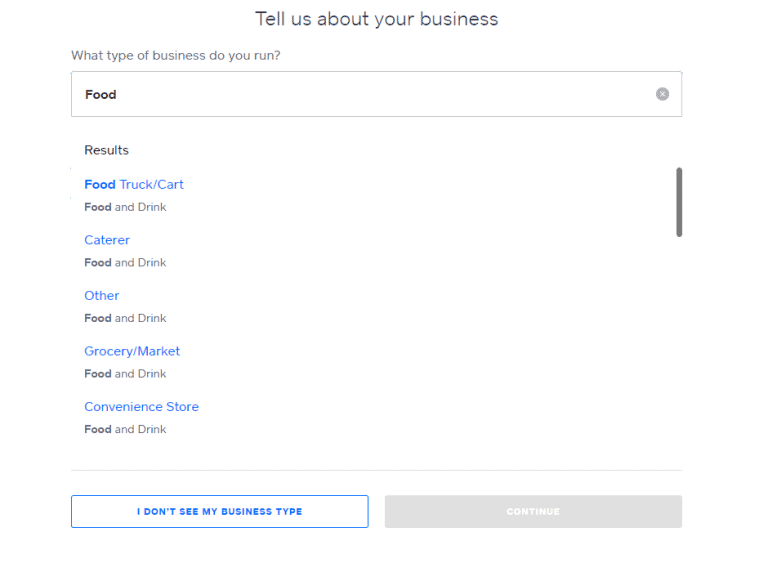The image displays a user interface form prompting the user to describe their business type. At the very top, gray text reads, "Tell us about your business." Below this, a question asks, "What type of business do you run?" inside a large rectangle where the word "food" is highlighted in black text. To the right of this search bar, there is an 'X' icon.

Beneath, a section labeled "results" presents various business categories. The first result, highlighted in blue text, reads "Food Truck - Cart," followed by the category "Food and Drink" in gray text. Next, "Caterer" is listed in blue text, again followed by "Food and Drink" in gray. Subsequent listings include "Other" in blue text with "Food and Drink" in gray, "Grocery - Market" accompanied by "Food and Drink," and lastly, "Convenience Store" paired with "Food and Drink."

On the left side, a blue-outlined rectangle contains the blue text, "I don't see my business type," indicating it as a clickable option. To the right, there is a long gray rectangle with the word "Continue" inside it, which is grayed out, suggesting it is not currently selectable. This implies that the user should choose "I don't see my business type" at this stage.